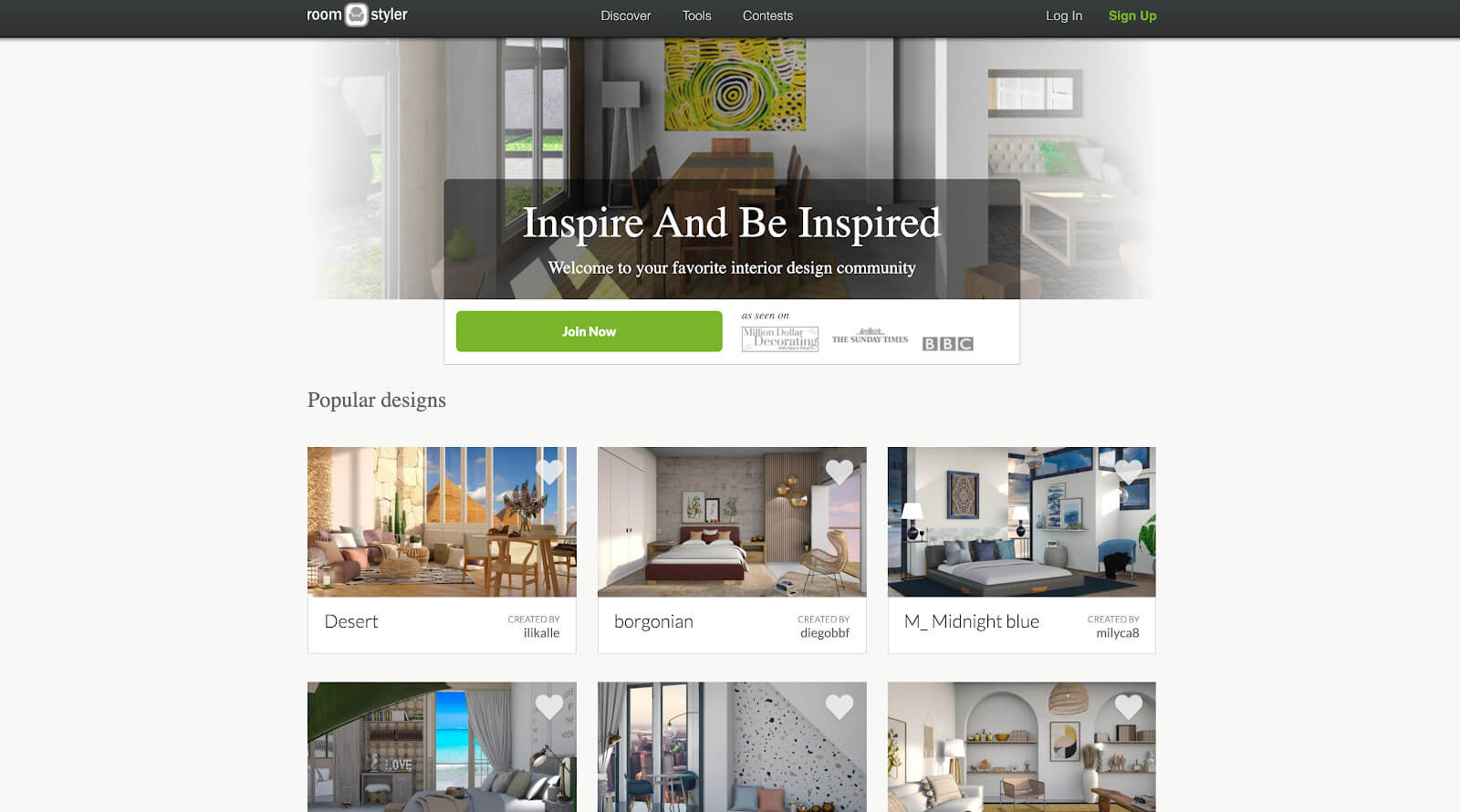This image captures a screenshot of a webpage on a computer, specifically from the Room Styler website. The webpage features the Room Styler logo prominently at the top, which includes an emblem of a chair between the words "Room" and "Styler." The navigation bar at the top of the page lists several options: "Discover," "Tools," and "Contest." 

To the right of the navigation bar, there are options to "Login" or "Sign Up," with the "Sign Up" button appearing in green for emphasis. The main section of the page features a welcoming message that reads, "Inspire and Be Inspired," followed by "Welcome to your favorite interior design community." It highlights the website's credibility by mentioning it has been featured on Million Dollar Decorating, The Sunday Times, and the BBC. 

Below the welcome text, there is a prominent call-to-action button, "Join Now," which is presented in a green, rounded rectangle with white text. 

Further down, the page displays a section titled "Popular Designs," showcasing several design entries. The first design shows a desert scene and is credited to "Created by Illacali." The second design, "Borgonian," is credited to "Created by Digogif." A third design, "M_Midnight Blue," is attributed to "Created by MillieCA8." Although the following images are cut off, it is apparent that users can like these designs as indicated by heart icons.